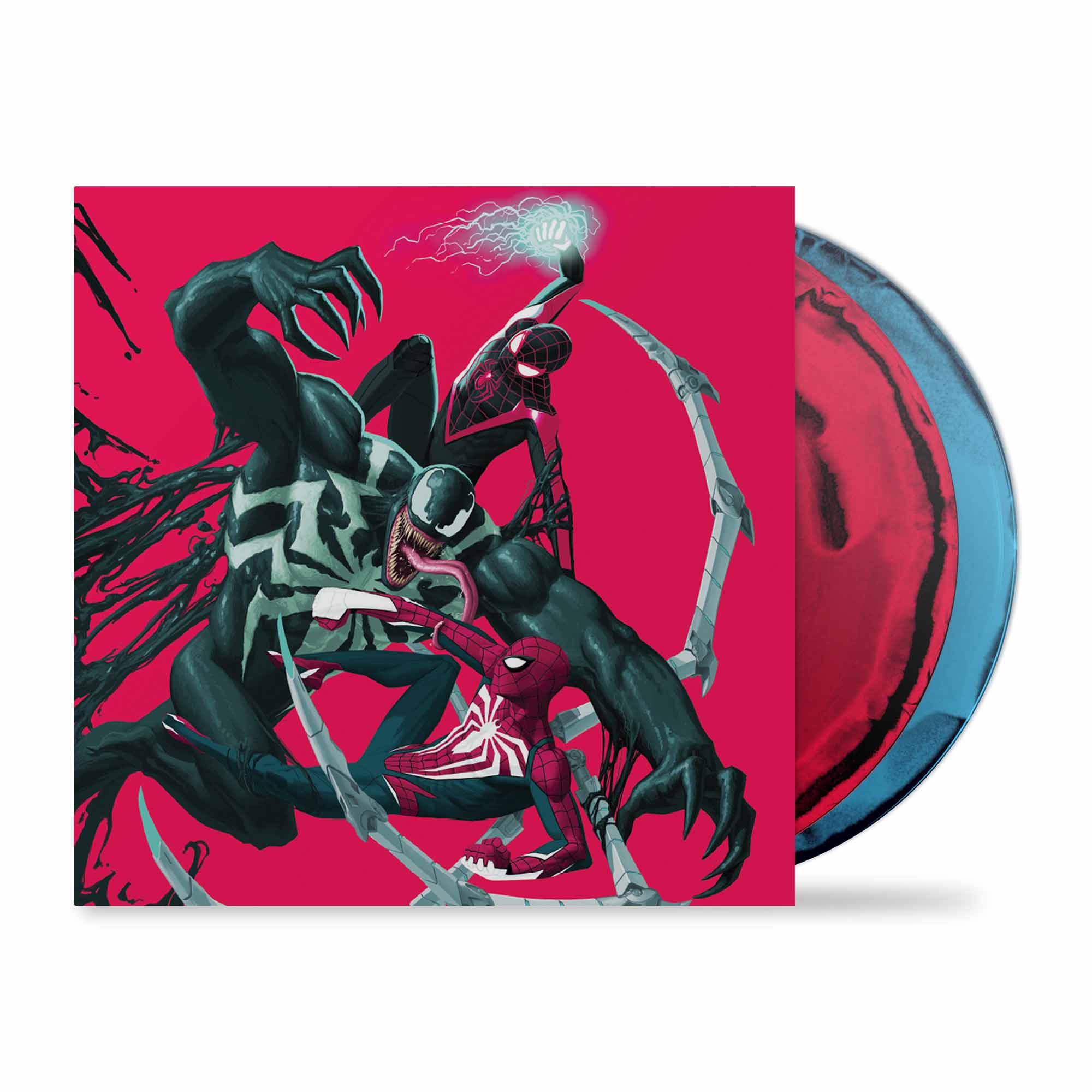The image showcases a colorful and dynamic scene on a square-shaped board that appears to be the cover of a CD package. The board, featuring a vivid red and pink background, is dominated by a dramatic battle involving multiple Spider-Man characters. Central to the scene is a villain, possibly Venom or a figure akin to Doc Ock, dressed in a black suit adorned with white designs and metallic tentacles emulating those on his chest. This villain is illustrated as the primary character, actively engaging in combat with two Spider-Man figures. One Spider-Man, clad in a black and red costume with a white spider emblem, is pictured kicking at the villain from a laid-back position. The secondary Spider-Man, potentially identified as Spin, is perched above, wielding a white flaming ball with streaming tails. In the background, black webbing or slime and robotic claws add to the intensity of the artwork. Behind the square board, partially visible, are two circular objects—one blue and the other red—against a stark white backdrop, providing a contrasting frame to the vibrant and action-packed centerpiece.